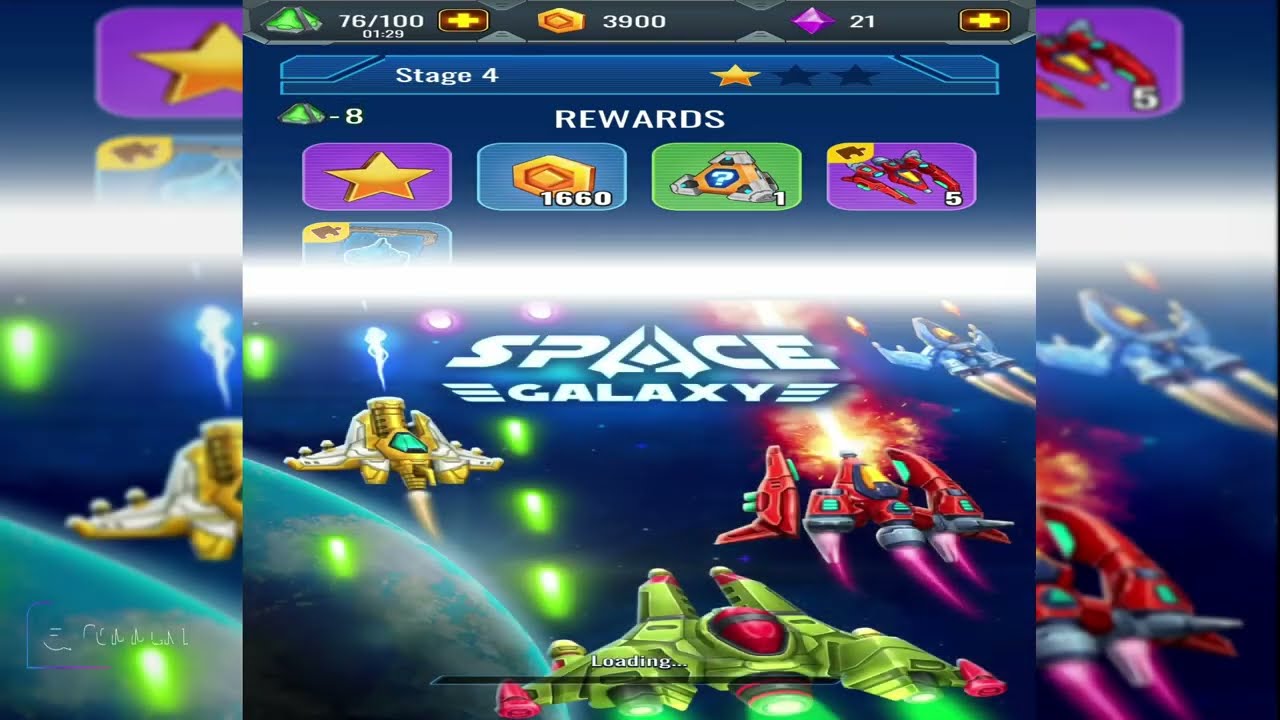The image is a detailed screenshot from the video game "Space Galaxy," depicting a loading screen combined with gameplay and control elements. Dominated by a space-themed backdrop with varying shades of blue, and featuring a partially visible green planet in the bottom left corner, the scene is vibrant and immersive. Several spaceships, colored red, blue, green, and yellow, occupy the bottom half of the image, each firing distinct projectiles: green bullets from the green ship, a whitish-blue laser from the yellow ship, a fire blast from the red ship, and yellow bullets from the blue ship. At the top, a banner adorned with stars sets off an array of reward boxes, each containing icons such as a star, a gold coin, a health cross, and a mystery box—these are brightly colored in green, blue, gold, and purple. The game's title, "Space Galaxy," commands the center of the image, while below it, text indicates the player is on Stage 4, having earned one out of three gold stars. A black loading bar at the very bottom, accompanied by the word "loading" in white text, suggests this is a transitional screen, possibly a wait screen before gameplay resumes. Overall, the scene is richly detailed, capturing the essence of a dynamic and colorful space shooter game.